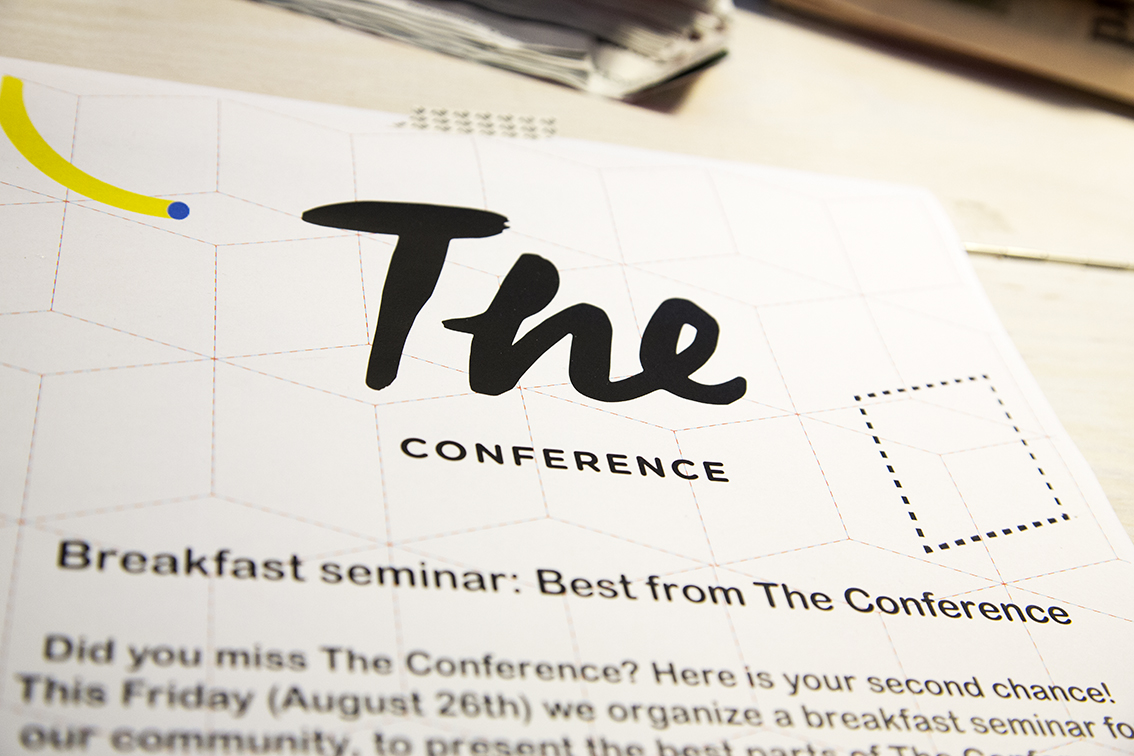The image is a rectangular photograph, wider from left to right than it is tall. It features a white piece of paper or pamphlet placed atop a white desk or table, taking up approximately 80% of the image's width. The background of the image is an off-white, with a section at the top displaying a black and brown frame-like structure, possibly a window or wall frame.

Dominating the center of the paper is a header where the word "THE" is written in cursive black ink, with "CONFERENCE" below it in a smaller, standard black font. Adjacent to this header, on the left side, there's a yellow swatch of color that curves around with a blue dot at the end. 

Beneath the main title, the text "BREAKFAST SEMINAR BEST FROM THE CONFERENCE" is printed in black. Below this, the following message appears: "Did you miss the conference? Here is your second chance. This Friday, August 26th, we organize a breakfast seminar for our community to present." However, the text fades off towards the bottom, making the rest of the message unreadable.

To the right of the main title and text, there is a black-dotted box, again containing several lines of text, and the lettering becomes indistinct as it descends toward the bottom of the page. Overall, the image conveys details about an upcoming breakfast seminar linked to a conference, presented in a clear and structured layout.